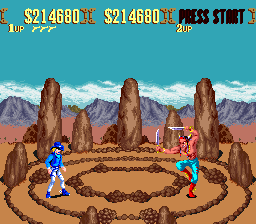In the middle of a desert landscape, this screenshot showcases an old arcade fighting game set in a circular stone arena. Surrounding the arena are tall rocks and mountains in the background. Atop the image, a score reads "$214,680" multiple times, indicating a close match with "ADD" and "University of California" also displayed. The arena itself features concentric circles of brown beads embedded in the stone ground. To the left stands a blue-clad cowboy, complete with a blue hat, shirt, and shoes. On the right is a shirtless Indian warrior with wings, holding two knives and wearing blue pants with red boots. His posture is dynamic, with one leg bent and the foot resting against the other straight leg. The scene is framed with arcade game elements like "Press Start," "1UP," and "2UP," suggesting active gameplay in a classic video game cabinet.